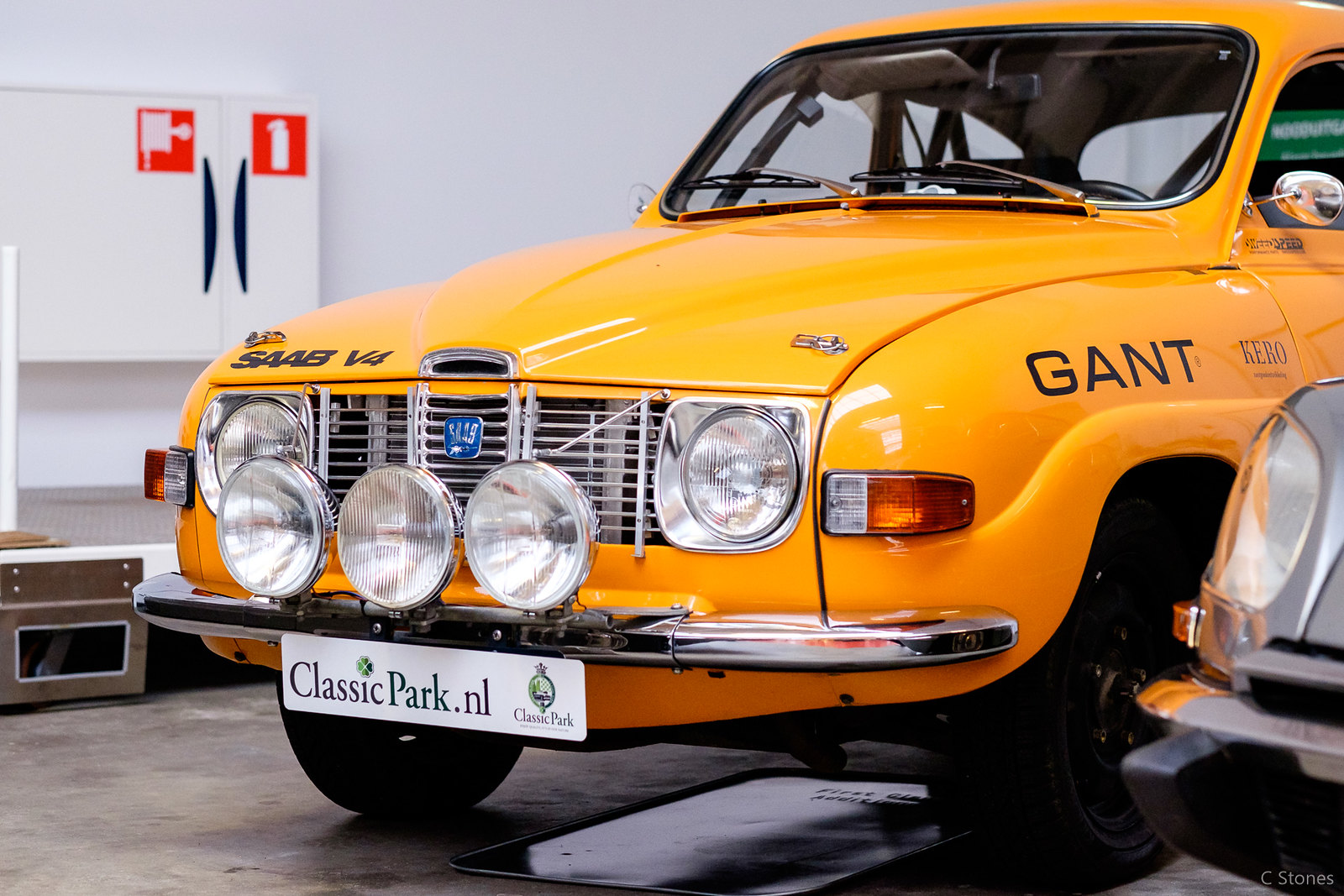The image captures a vibrant orange-yellow classic Saab V4 with meticulous detail. The car, showcasing a rounded front and left side up to the wing mirror, features five round headlights—two on each side and three centered on a chrome bar below a triangular-shaped silver grille with a blue emblem. The hood is marked with "Saab V4" in black, while "Gant" and "Kero" are inscribed above the front wheel arch. It has a white license plate displaying "classicpark.nl" accompanied by the Classic Park logo. Additional details include orange and clear front indicators, black tires, and silver mirrors. Positioned on a glossy reflective grey surface, the car is set against a white wall with cabinets and black handles, featuring a white fire extinguisher on a red background. A partially visible silver car appears in the bottom right corner, and the faint text "sea stones" is legible at the bottom.